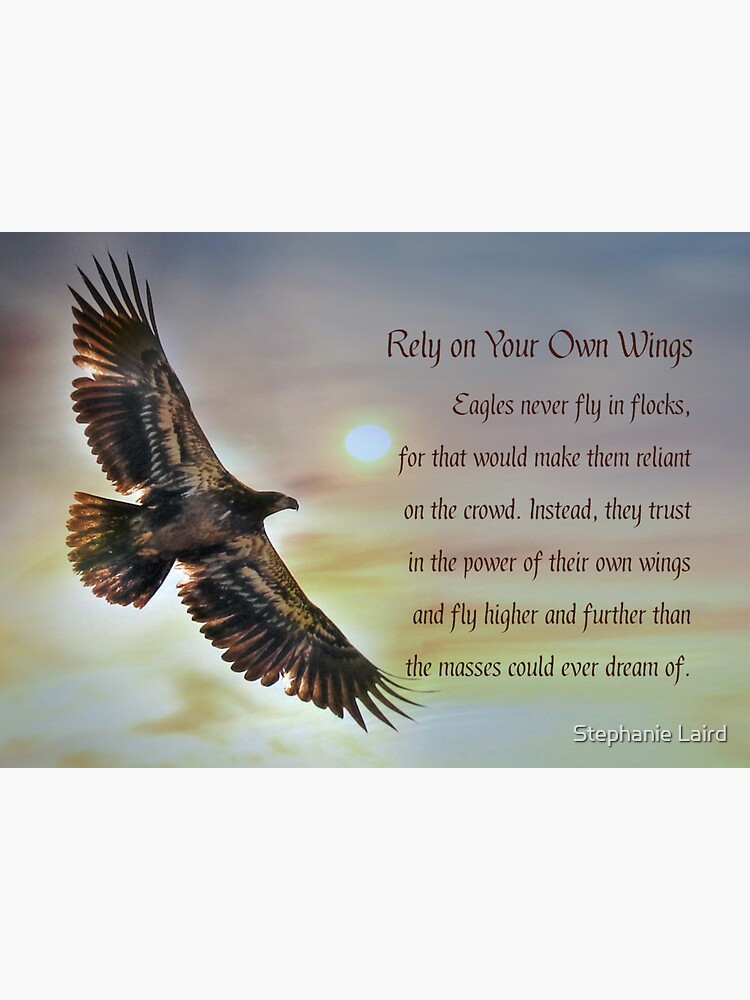This image is a small, approximately 7-inch wide by 5-inch tall poster featuring an uplifting scene. The background showcases a hazy sunset or sunrise with soft hues of yellow, light blue, and a touch of gray, along with some scattered clouds. 

Dominating the left-hand side, an eagle soars majestically with its wings fully outstretched. The eagle, rendered in naturalistic shades of brown, gold, and white, spans almost the entire height of the poster. Its tail feathers also spread out, and its head is turned towards the right. The intricate details make the eagle appear lifelike and powerful.

On the right-hand side, the text is displayed in a clear, elegant font. It reads: "Rely on your own wings. Eagles never fly in flocks, for that would make them reliant on the crowd. Instead, they trust in the power of their own wings and fly higher and farther than the masses could ever dream of." Below the inspiring quote, the author's name, Stephanie Laird, is printed in white text with capitalized initials.

The overall effect of the poster is highly motivational and positive, ideal for display in a space where one might desire a daily boost of encouragement.